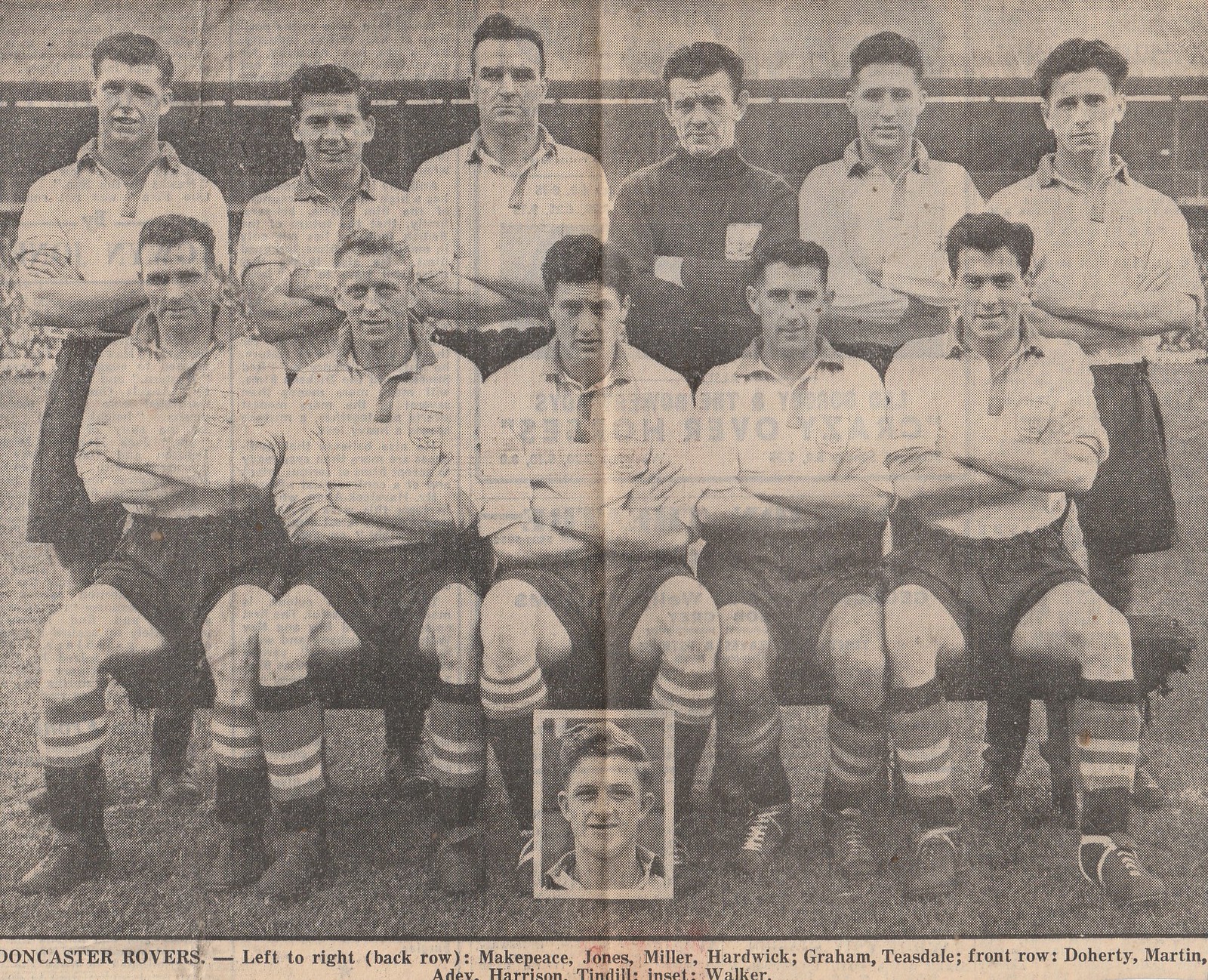This is an old, worn newspaper clipping that was once folded in half, with the crease line still visibly bisecting the paper. The clipping showcases a black and white photograph of the Doncaster Rovers football club. In the image, the team's players are arranged in two rows, with five players seated in the front row and six players standing in the back row. Below the photograph, there's a caption that reads "Doncaster Rovers," followed by "left to right" and then lists the names of the players. Curiously, there is an additional, separate picture of another player prominently placed in the center of the photograph, its purpose unexplained.